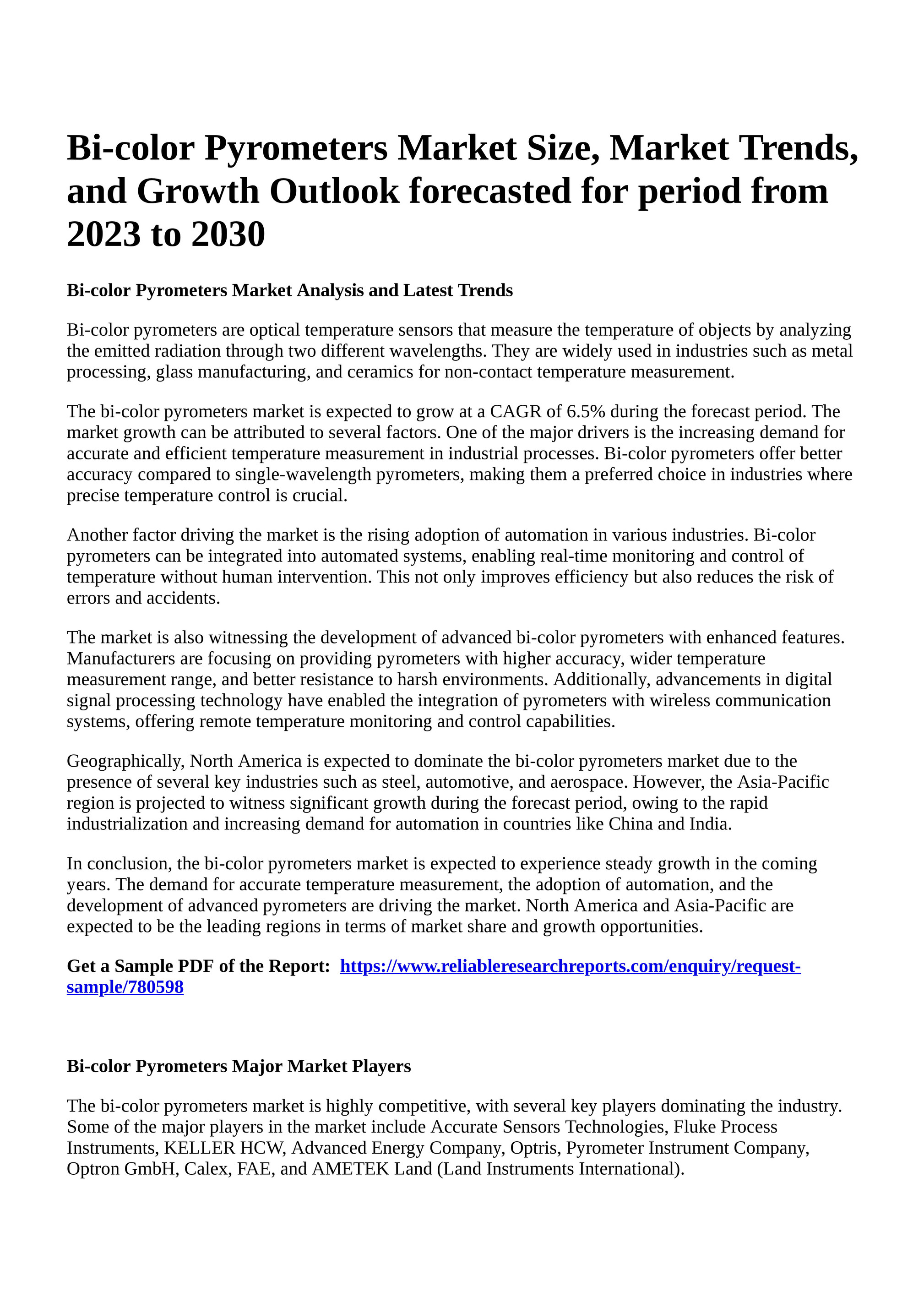The image depicts a detailed article with the prominent title boldly written at the top in black font, "By Color, Pyrometers, Market Size, Market Trends, and Growth Outlook Forecasted for Period from 2023 to 2030." The content, primarily focused on bicolor pyrometers, includes an analysis of market size, trends, and growth projections within this timeframe. The article is composed of six paragraphs, detailing the market analysis and latest trends. At the bottom of the text, readers are offered the opportunity to download a sample PDF of the report, with the link to the PDF highlighted in blue and underlined. Additionally, the article concludes with information about the major market players and further details, along with credentials of the author or editor. The overall format of the document suggests it is either a scientific or financial prognosticative paper, meticulously structured with sections of bolded and underlined text.